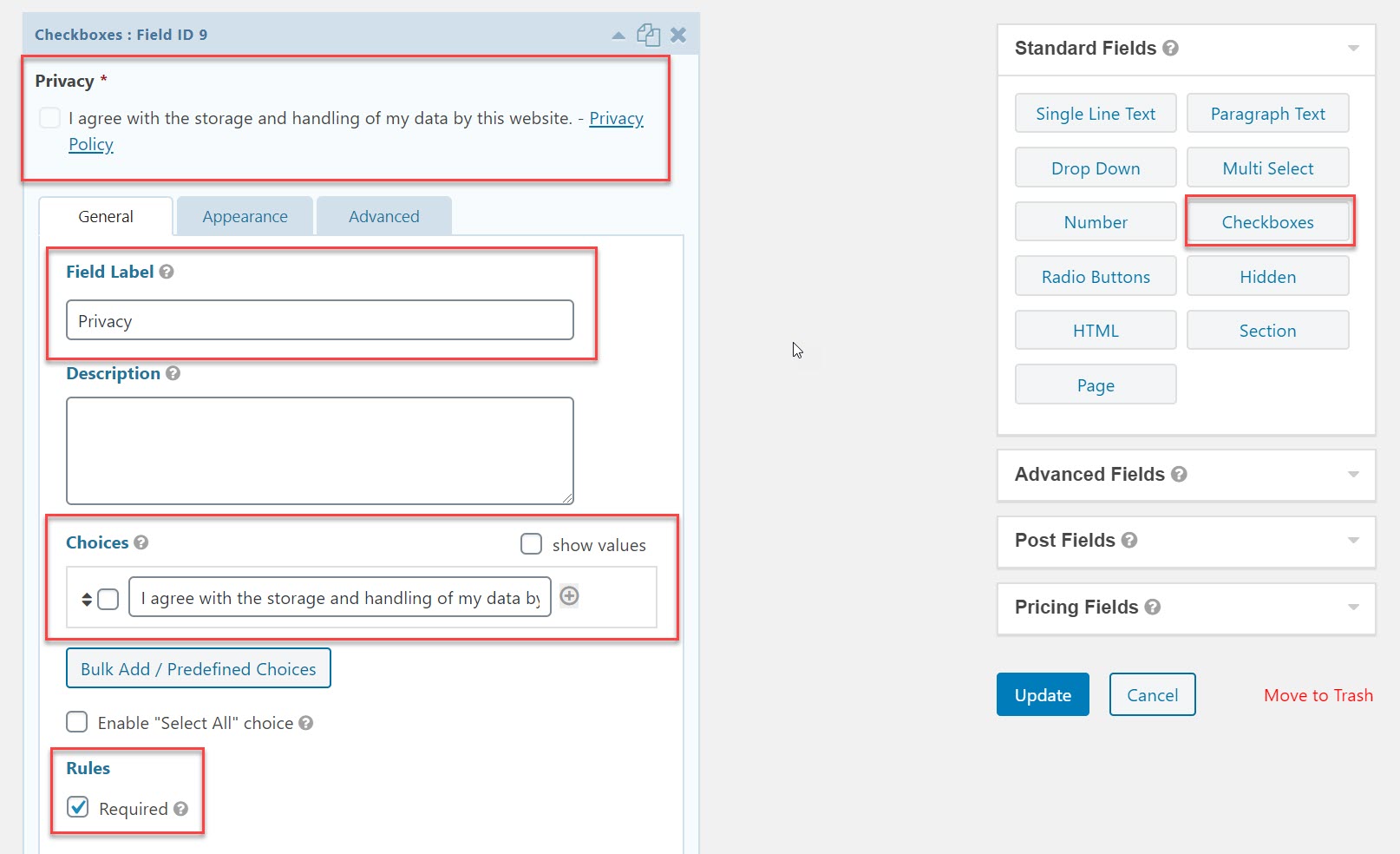The image depicts the setup process for adding a set of checkboxes to a user interface (UI). The interface is divided into two main sections: the left-hand side and the right-hand side.

**Left-Hand Side:**

At the top, a grayish-blue rectangle labeled "Checkboxes: Field ID 9" is visible. Adjacent to this label, icons include an upward triangle, two overlapping pieces of paper, and an X. Below it, there is a white background section titled "Privacy" with a red asterisk indicating a mandatory field. Inside this section, a checkbox labeled "I agree with the storage and handling of my data by this website" is present. Next to this, there is a blue link labeled "Privacy Policy," which redirects users to the privacy policy page. This entire area is highlighted with a red box, likely for emphasis.

Below this, there is another white section featuring three tabs: "General," "Appearance," and "Advanced." The "General" tab is currently selected. This tab contains various fields and options:

1. **Field Label:** Contains "Privacy" with a clickable question mark icon for more information.
2. **Description:** A text box with an adjacent question mark icon for additional details.
3. **Choices:** Accompanied by a question mark icon, and includes options like "Show values" checkbox, an agreement checkbox "I agree with the storage and handling of my data by," a plus sign, and a "Bulk add predefined choices" button.
4. **Enable Select All Choice:** A checkbox with a question mark icon.
5. **Rules:** A checkbox marked "Required" with a question mark icon.

The "General" tab fields for "Field Label," "Description," "Choices," and "Rules" are marked with a red box and are on a blue background, with labels in blue text and other informational text in black.

**Right-Hand Side:**

This section lists various fields under "Standard Fields" with an adjacent question mark icon for further details and a dropdown menu for additional selections. The available fields include:
- Single Line Text
- Drop-Down
- Number
- Radio Buttons
- HTML
- Page
- Paragraph
- Multi-Select
- Checkboxes
- Hidden
- Section

The "Checkboxes" option is emphasized with a red outline. Other menus titled "Advanced Fields," "Post Fields," and "Pricing Fields" are collapsed but have question mark icons next to them for more information when needed. 

At the bottom of this right-hand section, there are two buttons: an "Update" button, which is highlighted, and a "Cancel" button. Additionally, there is a "Move to Trash" link for deleting the current settings.

Overall, the image shows a detailed UI configuration setup where a user is adding checkboxes and configuring various fields and options to manage privacy-related data.